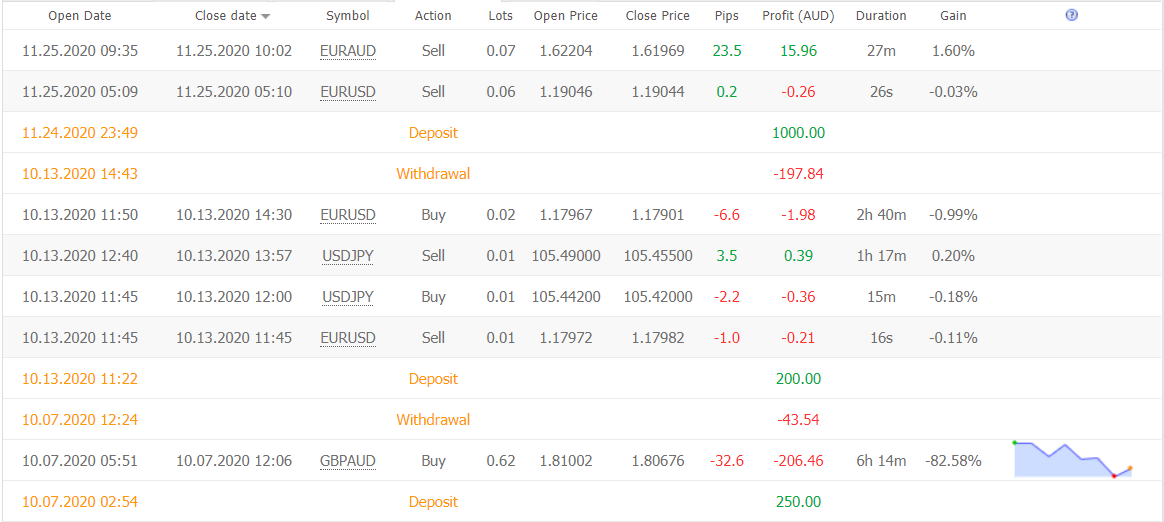A screenshot of a computer display showcases a detailed spreadsheet set against a predominantly white background. The spreadsheet features rows of data, with alternating white and gray lines for easier readability. At the top of the screen, column headers are clearly visible, starting from the left with "Open Date" and progressing rightwards to "Close Date," followed by "Symbol," "Action," "Lots," "Open Price," "Close Price," "Pips," "Profit (USD)," "Duration," and "Gain." In the lower right-hand corner, a line graph provides a visual representation of financial performance, likely related to stocks or bonds, offering an analytical view of the data trends. The dataset includes dates predominantly from October and November 2020, reflecting the period under analysis.